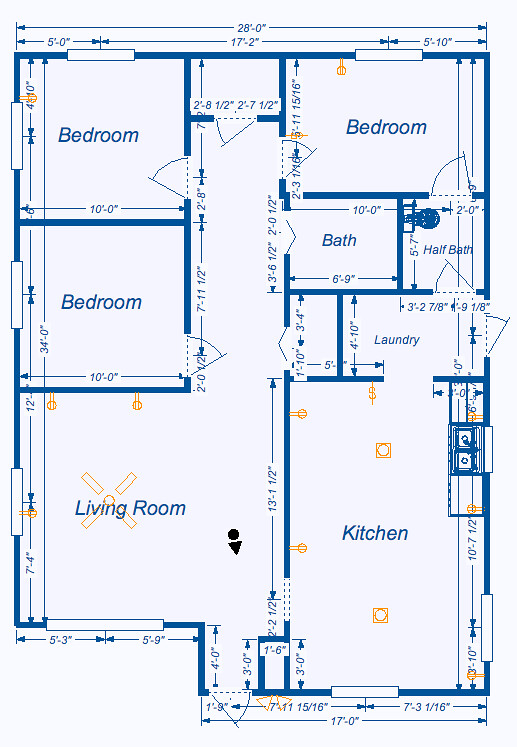This image depicts a detailed blueprint drawing of a house layout. Starting from the top, the blueprint indicates a width of 28 feet, with a centered arrow spanning this distance. From the center point, there is a 5-foot measurement extending to the center of the first window, followed by a 17.2-foot span to the center of the next window, and then 5 feet 10 inches from this window center to the adjacent wall.

On the left-hand side, there is a bedroom labeled with blue text indicating it measures 10 feet. This bedroom contains an interior window. Directly below this first bedroom, there is another bedroom also measuring 10 feet. A 34-foot-long wall runs from these two bedrooms all the way to the living room area.

The living room features a prominent black circle, possibly indicating a fixture or a focal point, and points towards a door. Adjacent to the living room are the kitchen, laundry room, and a half bath that connects to another bedroom. This second bedroom leads into a hallway, which includes an additional bathroom with an attached closet.